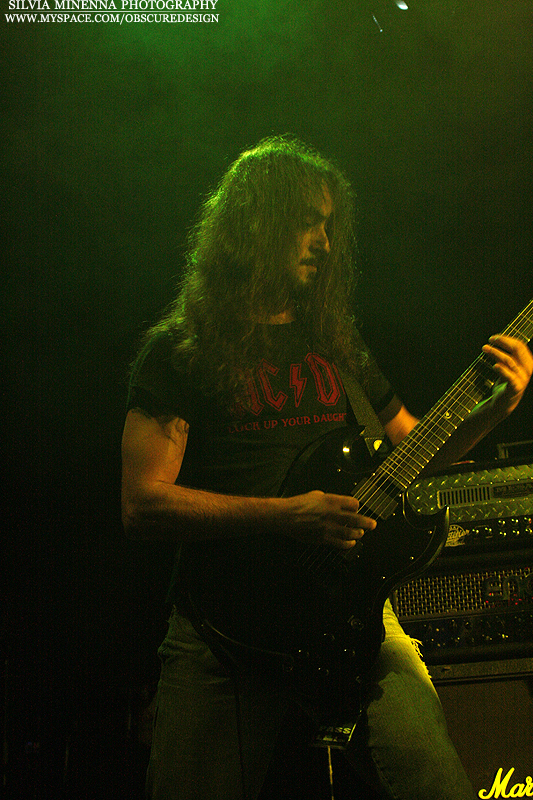In this vertical photograph, a Caucasian gentleman with long hair and a goatee stands at the center, energetically playing a black Gibson SG electric guitar. He is wearing frayed blue jeans and a black ACDC t-shirt adorned with red lettering. The setting is a dark concert venue, enhanced by smoky effects and subtle orange lighting, which contrast sharply with the focused spotlight illuminating him. Behind him, multiple amplifiers are visible, prominently featuring a Marshall amplifier with partial lettering ("M-A-R") in yellow font in the lower right-hand corner. The photographer's information, "Sylvia Manetta Photography," along with her social media handle, "www.myspace.com/obscuredesign," is positioned in the upper left-hand corner of the image, indicating the origin of this striking and atmospheric live performance capture.